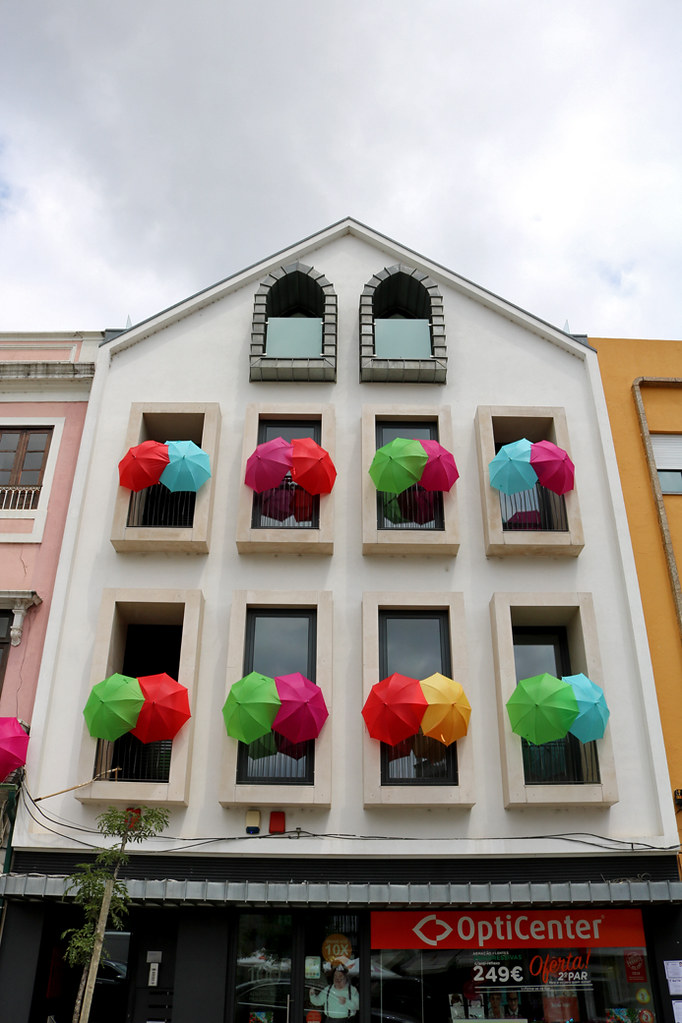This color photograph captures an exterior view of a four-story building, combining commercial and residential spaces, likely located in England as suggested by the currency symbol "pounds" on the signage. The building has an A-shaped, peaked roof and is part of a connected series of structures, presenting a townhouse style. 

The top floor features two arched windows, each partially covered with window shades. These windows are framed in gray stone, contrasting with the white facade of the upper portion of the building. Below the attic windows, there are two rows of rectangular windows, with each row comprising four windows. The top row is slightly shorter than the bottom row. 

In total, there are sixteen multicolored umbrellas—two per window—protruding from these lower windows. The umbrellas display a vibrant array of colors, including red, light blue, purple, green, yellow, teal, and orange. 

The ground floor of the building houses a commercial establishment named "OptiCenter," indicated by a prominent red sign in the front window, which also displays the number "249" and a "two pair" offer. The storefront suggests it is an optical center, and there is a power line draped along the bottom edge of the upper white portion of the building. Additionally, the image captures a Caucasian man standing in the doorway of the ground floor, further adding to the detailed urban scene.